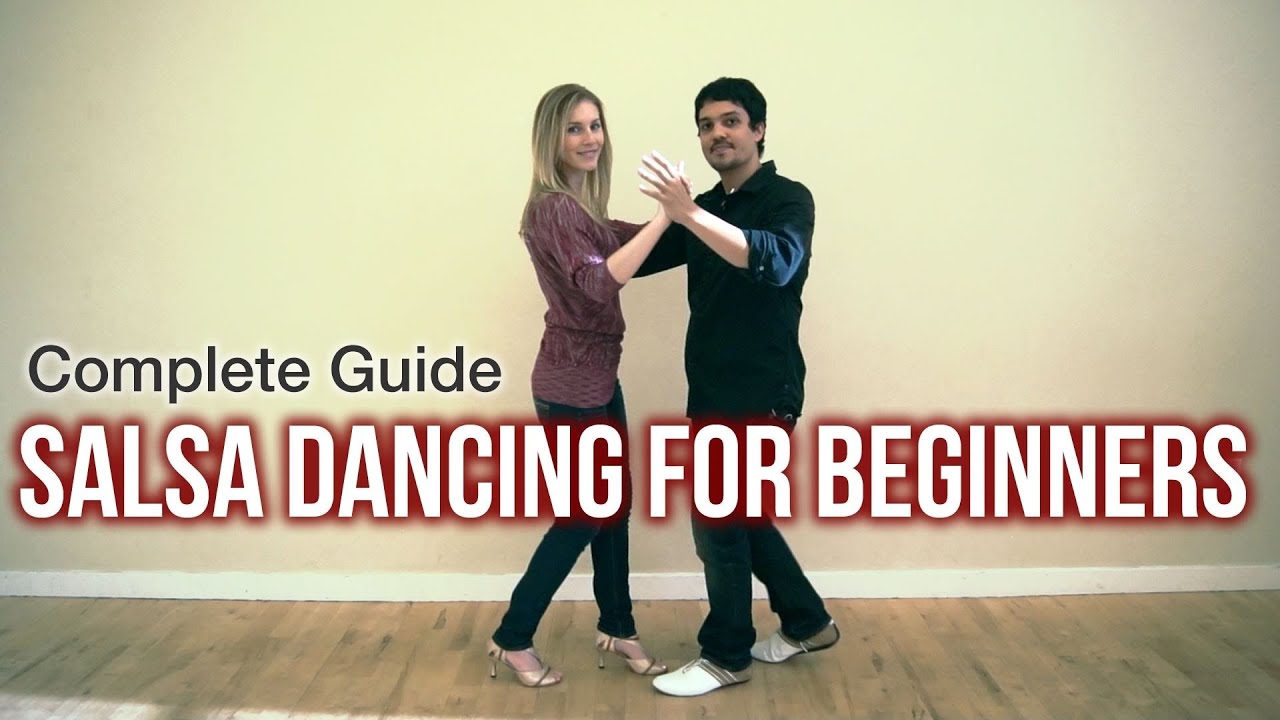This landscape-oriented photograph captures a moment of a couple dancing on a hardwood floor. The man, who stands on the left, appears to be in his thirties, with brown hair, a mustache, and a bit of a beard. He is dressed in a dark shirt, dark jeans, and white shoes reminiscent of golfing shoes. His left arm is raised, clasping the right hand of a slender woman to his left. She has long, dirty blonde hair and is wearing a long, plum-colored tunic with long pants and high-heeled gold shoes. The couple is looking directly at the camera and smiling, while a beige wall with white baseboard trim serves as the backdrop. Across the top of the photograph, the text reads "Complete Guide to Salsa Dancing for Beginners," with "Complete Guide" in black letters and "salsa dancing for beginners" in white letters on a red background.